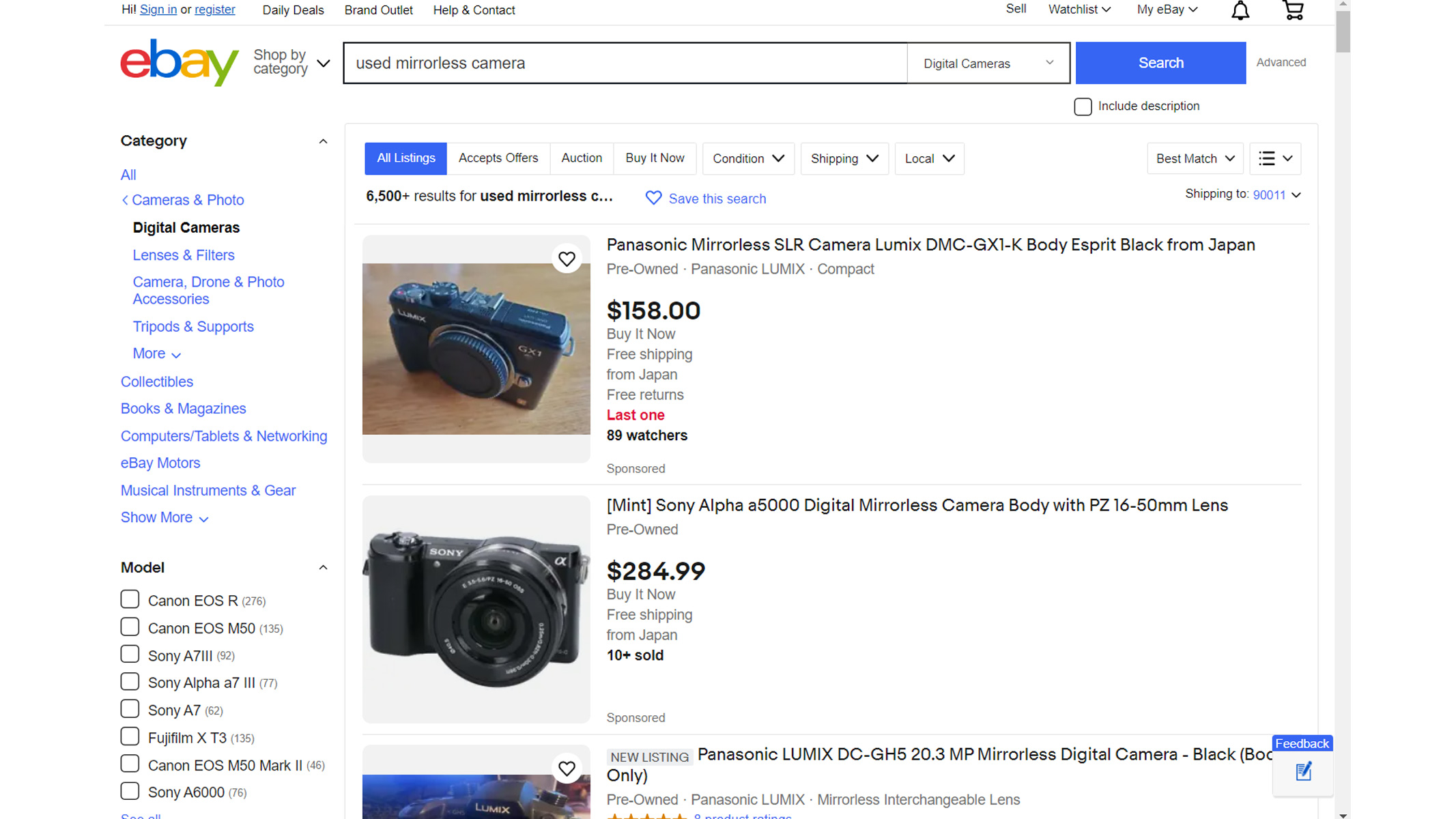At the upper left corner of the interface, the word "Hi" is displayed, followed by options to either "Sign Up" or "Register". Below these options, the eBay logo is prominently featured, with the letters "E" in red, "B" in blue, "A" in yellow, and "Y" in green. Adjacent to the logo is a long search bar containing the placeholder text "Search", with a blue square button to its right labeled "All Listings".

Displayed below is a listing for a camera, featuring an image of a basic black camera with its lens cap on. The description reads "Panasonic Mirrorless SLR Camera, Lumix DMC Body E-Spirit Black from Japan" and the price is marked at $158. The phrase "Last One" is highlighted in red. Below this is another listing for a camera, this time a "Sony Alpha Digital Mirrorless Camera with PZ 16-50mm Lens," priced at $284.99.

The third listing partially shows the top of a camera, but the description is visible: "Panasonic Lumix DC GH5 20.3 MP Mirrorless Digital Camera Black Box." At the upper right of the interface, icons for a bell and a shopping cart are displayed.